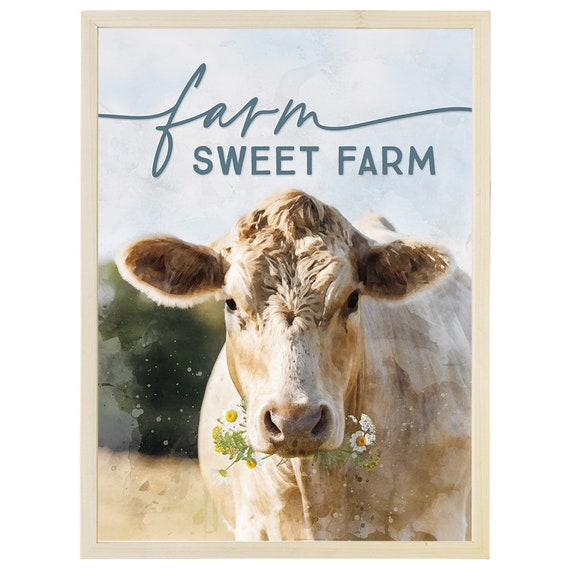The image is a tall rectangular portrait with a thin, white-brown border framing it. At the center, a cow faces directly toward the viewer. The cow is primarily off-white with light brown patterns across its fur, and its medium-brown ears stick out to the sides. The top of its head is also a lighter brown. In its mouth, the cow holds two types of flowers: white flowers with yellow centers on the left and yellow flowers on the right. Over the cow's head, in front of a bright blue sky with light cloud cover, the words "Farm Sweet Farm" are written in medium blue cursive. Below the cow, there's a dark green gradient area, possibly representing abstract grass or dirt, creating a serene, rural atmosphere. The overall image is characterized by its soft, neutral colors and gentle brush strokes, evoking a calm, homey, and relaxed feeling, reminiscent of quiet country farm life.